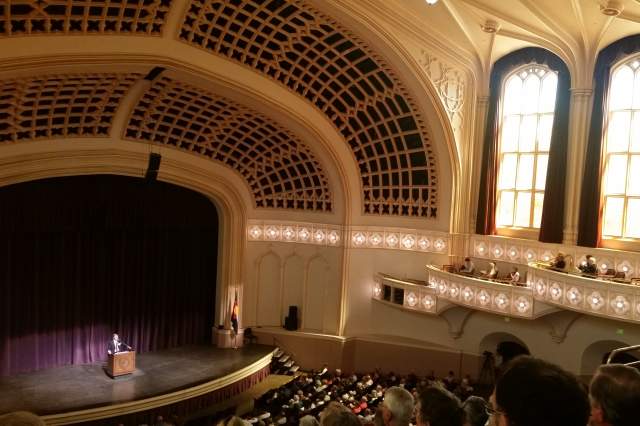The image depicts the interior of a grand, historical auditorium, viewed from the upper left-hand corner, high up in the seating area, possibly from the balcony. Centrally positioned on the stage, a person stands at a brown wooden pulpit, speaking into a microphone. The stage is framed by very tall, closed velvet curtains in purple, providing an elegant backdrop. The auditorium features an intricately decorated beige-colored archway overhead, enhancing its church-like yet theatrical ambiance. 

To the right-hand side of the stage stands a flag, likely a German flag, and a spotlight illuminates the speaker. The audience fills the seats completely, as well as the side theatre boxes. These boxes, or VIP sections, are adorned with lights and are positioned beside two enormous arched windows draped with dark brown curtains, through which sunlight softly filters in. The entire scene suggests a setting suited for operas, stage presentations, or formal lectures.